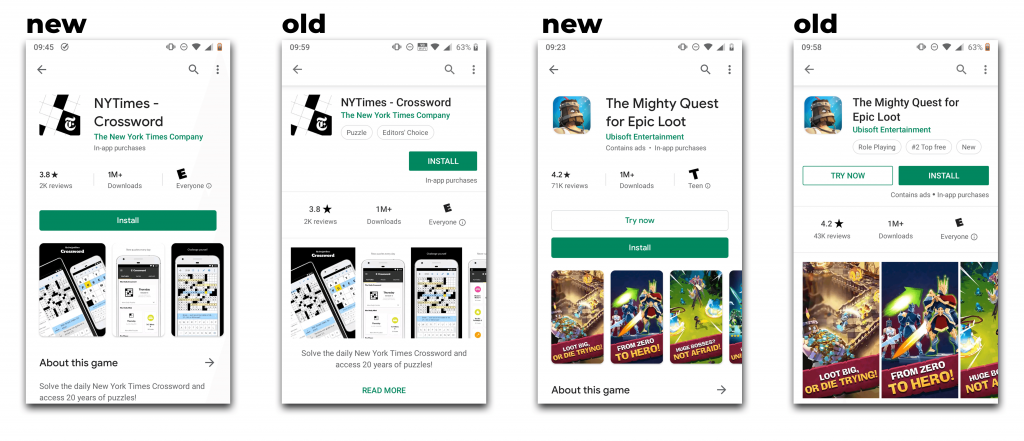This image consists of screenshots from a cell phone, depicting a comparison between old and new designs for app store listings. There are four images arranged from left to right, showcasing two different apps. 

On the far left, the New York Times Crossword app is highlighted. The first image shows the older design, with a smaller "Install" button, under the label "old" in black letters. Next to it, the updated design is displayed, featuring a larger "Install" button and labeled as "new."

The two images on the right focus on the game "The Mighty Quest for Epic Loot." The first shows the older design, with smaller "Try Now" and "Install" buttons. In contrast, the updated design next to it features enlarged "Try Now" and "Install" buttons that appear smoother and more visually appealing.

Overall, the redesigned app store listings highlight larger, more user-friendly buttons for both the New York Times Crossword and The Mighty Quest for Epic Loot apps.